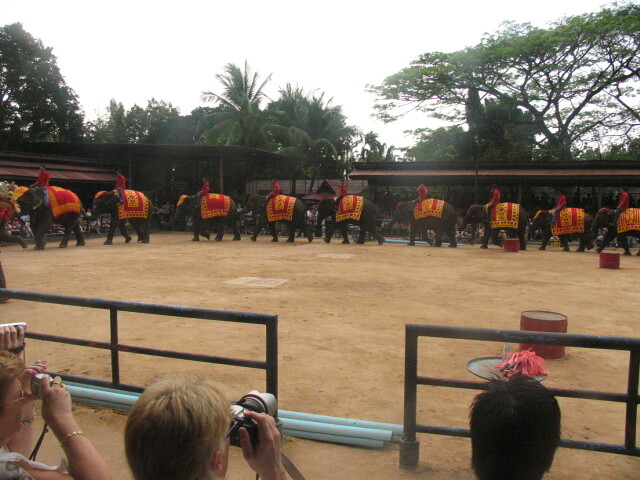In this captivating outdoor scene at an elephant park or zoo, a small arena hosts an engaging elephant show. The arena's light brown dirt floor is adorned with three red barrels, possibly part of the performance. Eleven majestic, deep gray elephants walk in a circle, each trunk holding the tail of the elephant ahead, forming a unified and graceful procession. These elephants are elegantly dressed in decorative gold and red jackets with matching red and gold headdresses, topped with striking red feather plumes.

In the foreground, only the backs of three spectators are visible. The two women on the left are actively snapping pictures of the mesmerizing scene, while the person on the right, sporting short dark brown hair, calmly observes the spectacle. The arena is flanked by covered pavilions with dark brown roofs, adding a rustic charm to the setting.

Beyond the arena, a dense backdrop of trees creates a lush, verdant perimeter. The trees enhance the natural beauty of the location while indicating that the event is taking place in an exotic and possibly tropical locale. The sky above is overcast with thick clouds, suggesting imminent rain, which adds a dramatic element to this otherwise lively and colorful spectacle.